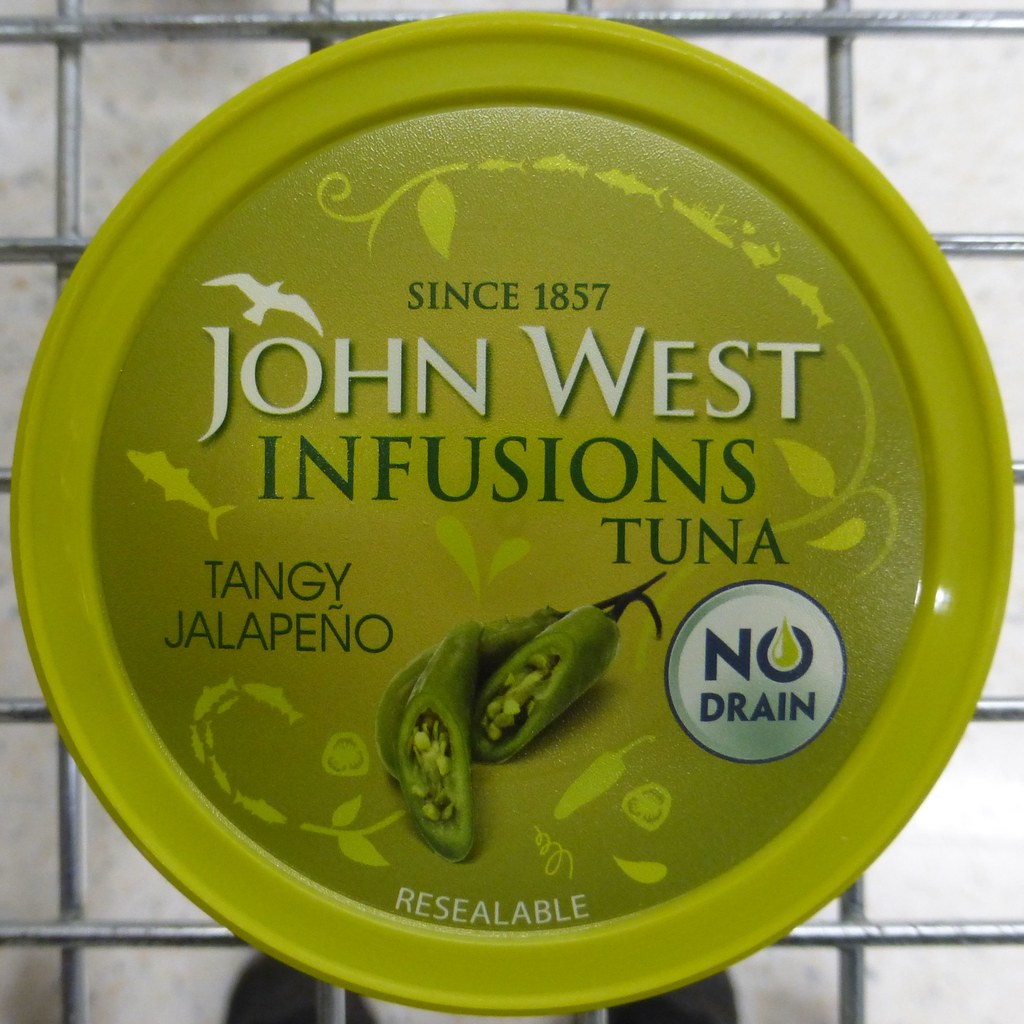The image features the top view of a green, round, plastic container placed on a metal cooling rack or the bottom of a shopping cart. The container is labeled with a green and white sticker that prominently displays the brand "John West Infusions Tuna" and emphasizes its "Since 1857" heritage. The flavor is described as "Tangy Jalapeno," and it notes that the container is "Resealable" and requires "No Drain." The label is adorned with detailed illustrations of jalapenos, including three prominent peppers in the center, two of which are sliced open to reveal their seeds. Additional design elements include outlines of jalapenos and tunas, as well as a whimsical depiction of a tuna chasing smaller fish beneath a boat. The limey olive green container has dented edges, and the vibrant colors draw attention to its unique packaging.